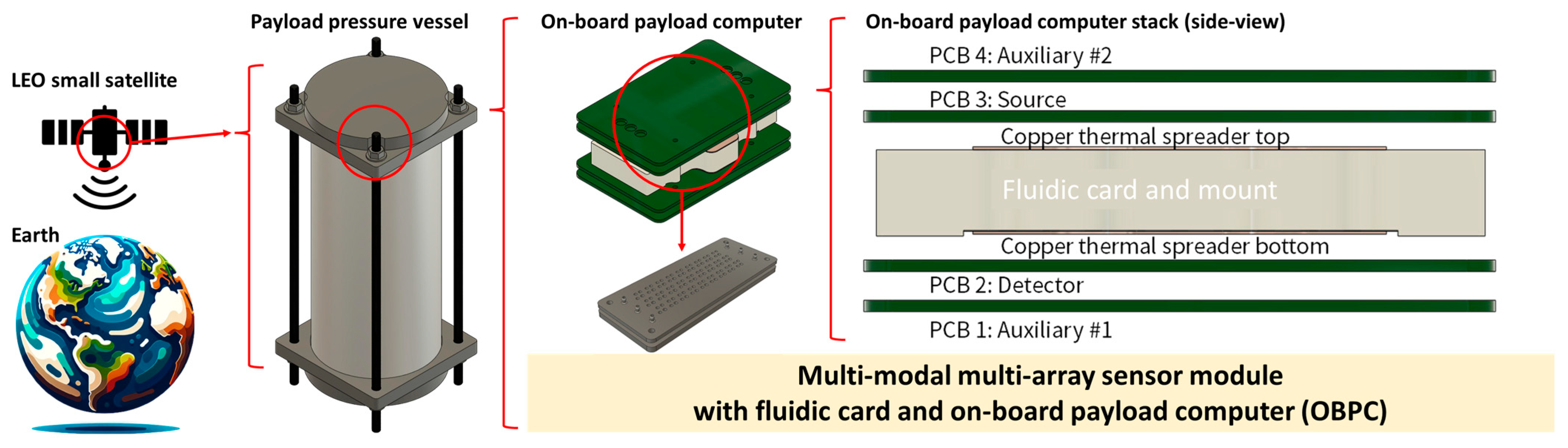The image is a detailed color diagram depicting a multimodal, multi-array sensor module with a fluidic card and an onboard payload computer (OBPC), shown to be part of a Low Earth Orbit (LEO) small satellite system. Starting from the left, the diagram illustrates an LEO small satellite orbiting Earth, characterized by wave bars indicating its communication path. Adjacent to this is an illustration of the payload pressure vessel, a cylindrical component held together by tubes. In a yellow, elongated box with black bold letters towards the bottom right, the diagram explicitly labels the OBPC. To the right, a detailed stack side view of the OBPC reveals various components including PCB4 auxiliary number two, PCB3 source, a coupler thermal spreader top, and a fluid card mount. Each of these detailed parts, highlighted in green, exemplify the intricate layering of the onboard payload computer, which is pivotal in the satellite's operation.